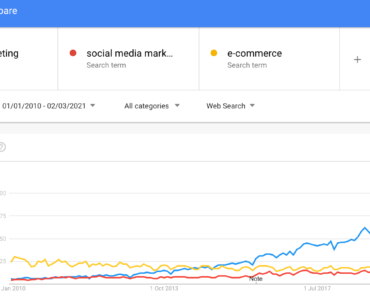The image showcases a detailed analytical chart with a blue border at the top, featuring the label "Social Media Marketing" highlighted by a red circle. Additionally, it includes search terms such as "e-commerce" marked by a yellow dot. The date range indicated spans from January 1, 2010, to February 3, 2021, with corresponding dropdown menus for query refinements including "All Categories" and "Web Search."

The chart is segmented by gray lines and a lighter gray border, each denoting various data points: 80, 75, 60, and 25. A trio of colored lines representing different data trends traverse the chart. The yellow line commences at the 25 mark, the red line starts at 0, and they converge towards the right-hand side. Meanwhile, the blue line mirrors the red line initially but concludes at 65 towards the right.

Key dates annotated along the bottom axis include January 2019, October 1st, 2019, and July 1st, 2017, providing temporal context for the data trends represented by the colored lines.